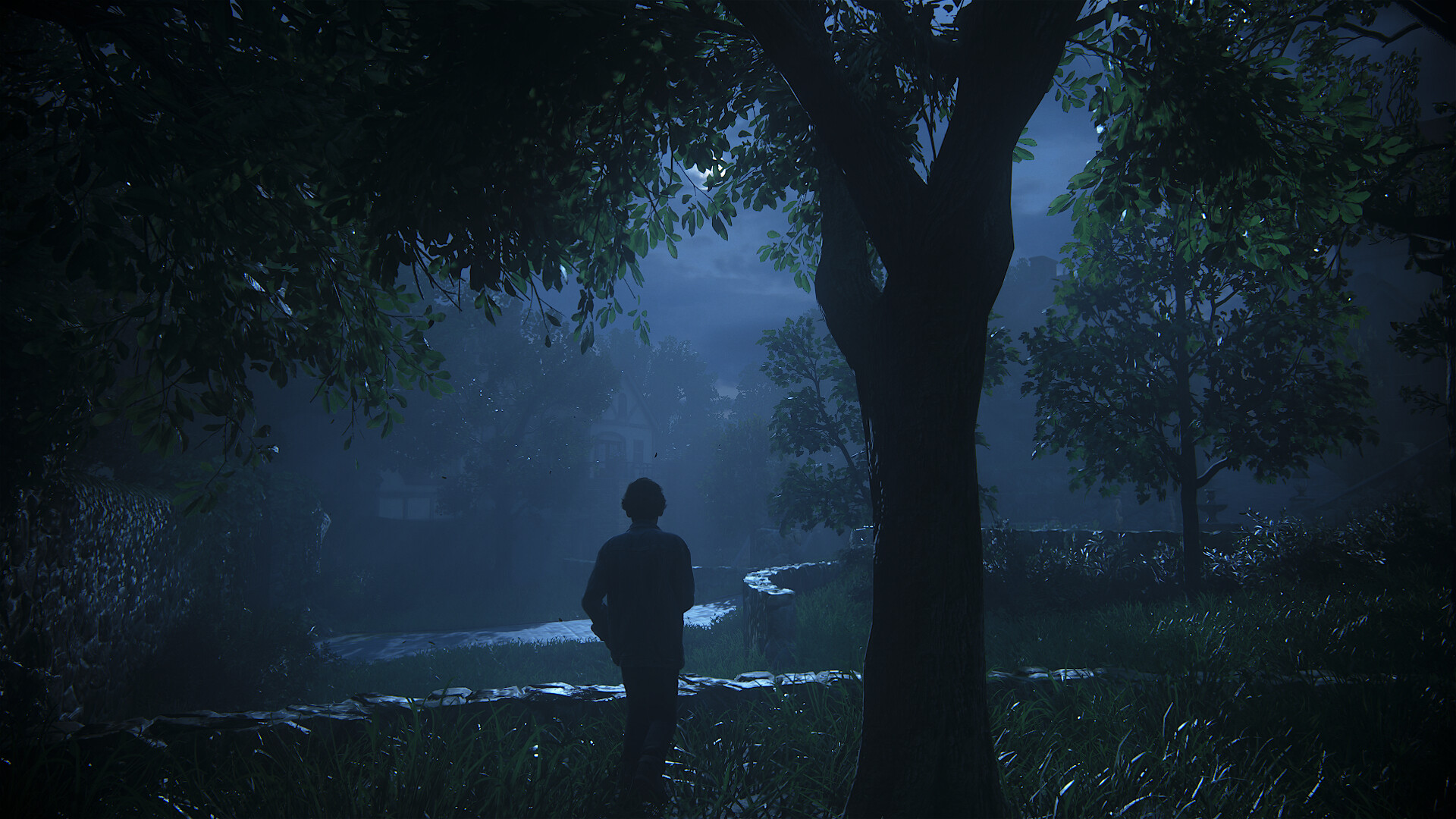In this captivating scene reminiscent of a video game, the sky is dominated by a luminous full moon casting a mesmerizing white light, creating an ethereal glow that accentuates the serene nighttime atmosphere. Shades of deep blue permeate the sky, blending into the moonlight, while subtle beams of light cascade downwards, illuminating the landscape below in a gentle, otherworldly radiance.

The top of the image is adorned with verdant green leaves that frame the scene like a natural canopy, while the bottom showcases more greenery that transitions smoothly into rugged stone formations. At the heart of this tranquil setting stands a solitary figure cloaked in black shadow, gazing contemplatively at the surroundings, adding a touch of mystery to the tableau.

A majestic tree dominates the center of the image, its robust bark providing a strong focal point. To the right, an explosion of green foliage further enhances the lushness of the scene. In the background, a quaint house emerges from the shadows, its walls constructed of pristine white wood. Several windows are visible, hinting at life within and adding a final touch of homely comfort to this richly detailed image.